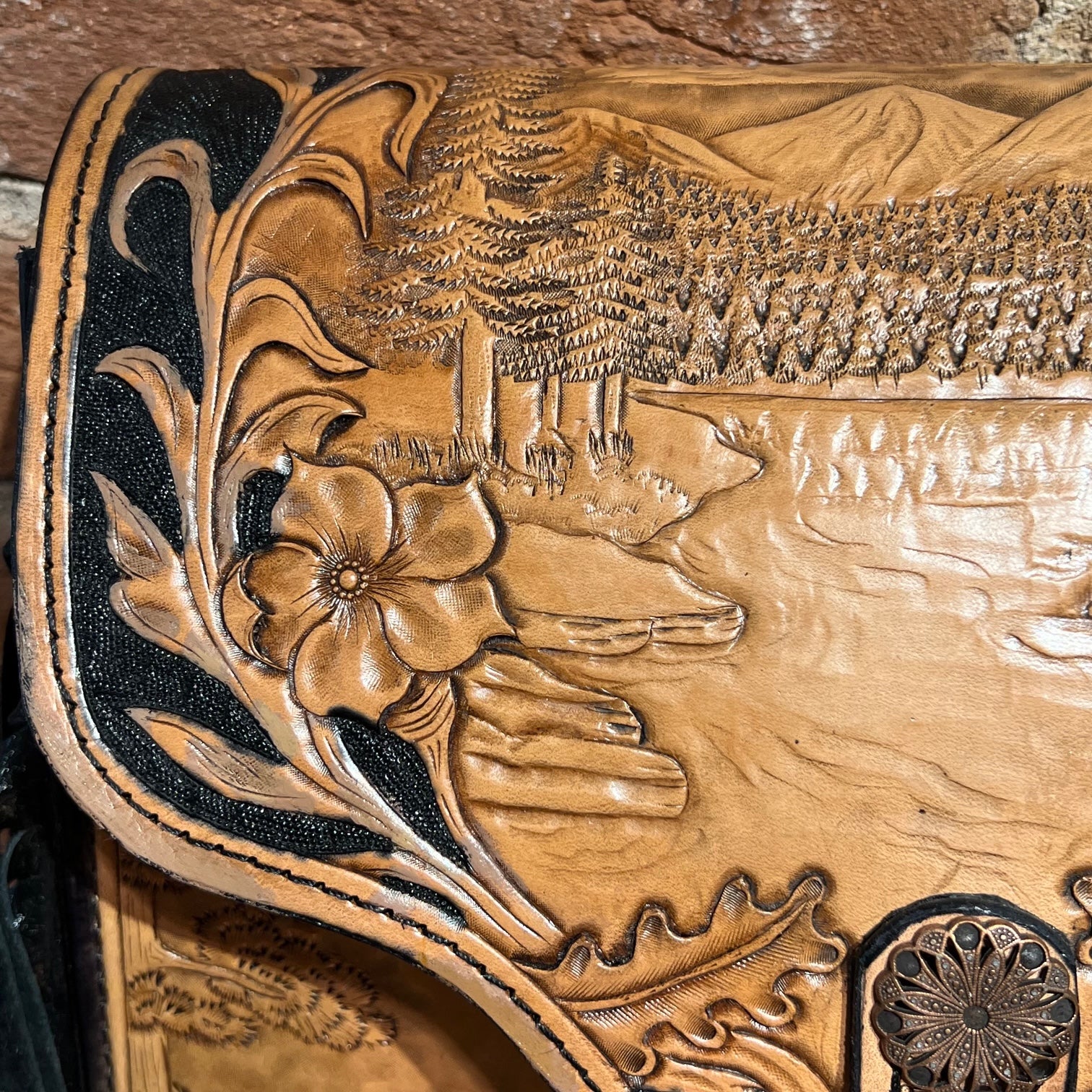The image captures a close-up view of a leather piece with detailed engravings. The leather, possibly a holster, bag, or saddle, features intricate designs that suggest a natural scene. The material appears to be a kind of processed, possibly plasticky leather, trimmed in black. Engraved on the surface is a landscape depicting long fields of evergreen trees, a body of water with visible ripples, and a range of mountains shaded in two tones of brown to accentuate their elevations. The leather also showcases smaller details, such as stems with leaves and flowers—one flower with five petals and a circular center, and another spiral, flower-like motif colored in black. The grooves of the engravings are filled with black to create a textured appearance. The background in the image is out of focus, revealing only a hint of brown wood behind the leather piece, emphasizing the complex and artistic craftsmanship of the leatherwork.